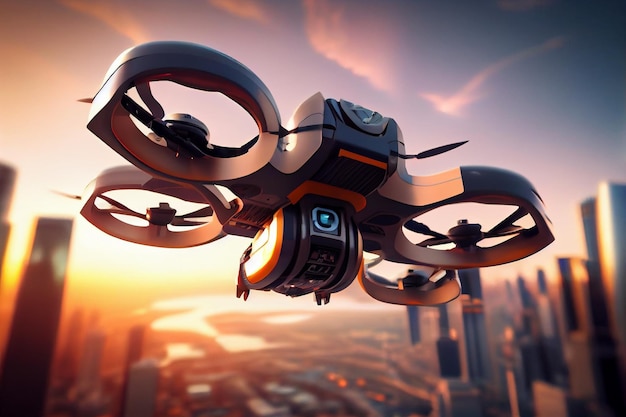In this detailed, digitally-rendered image, a futuristic drone hovers over a sprawling, metropolitan cityscape at sunset. The drone features a sleek, modern design with four circular propellers, two on each side, and a combination of black, white, and orange tones. A blue camera, housed within a semi-circular area on the drone's underside, suggests surveillance capabilities. The sky is awash with the warm hues of a setting sun, blending vibrant oranges, pinks, and purples with wisps of light blue clouds. The city beneath, reminiscent of New York City, is filled with towering skyscrapers with reflective glass facades and scattered shorter buildings. In the distance, a body of water possibly an inlet or a lake, adds depth to the scene, enhancing the image's futuristic ambiance. The overall composition suggests a highly advanced urban environment, embodying a vision of a distant future.